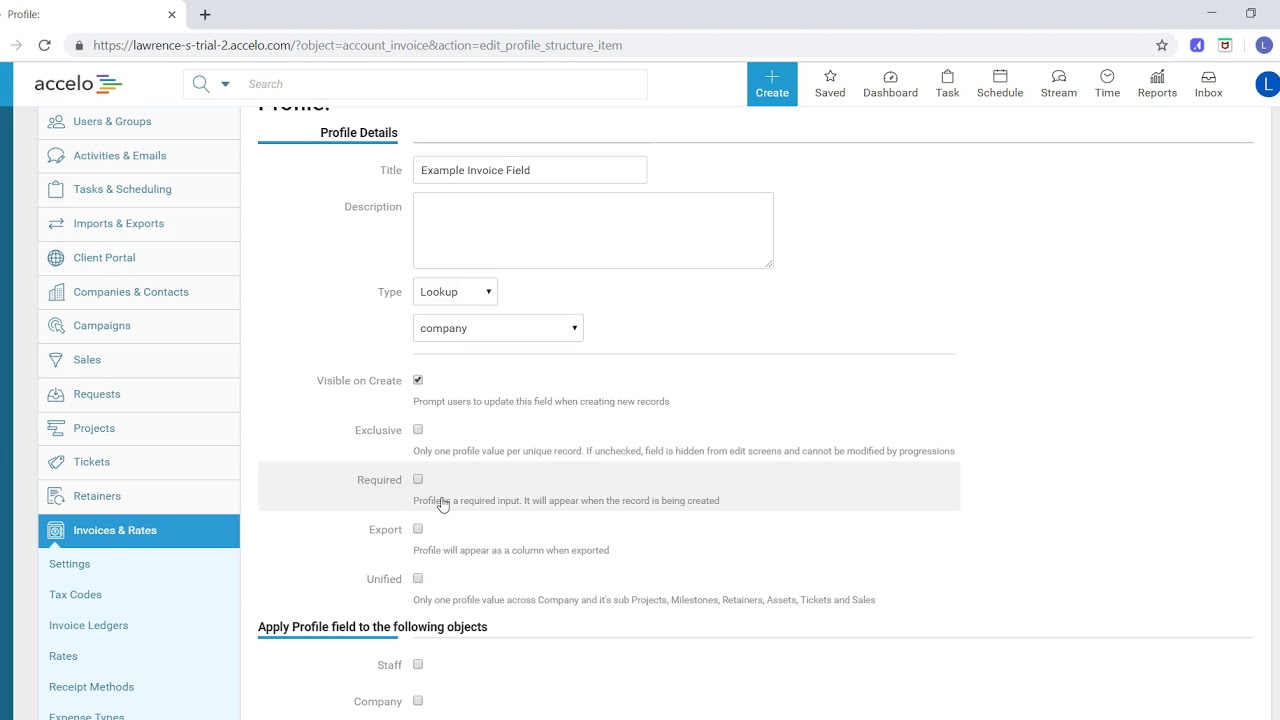The image displays a detailed interface of a project management software, showcasing various elements and navigation options. At the top, there's a navigation bar with icons and text including "Profile," "Square Bar," and "Refresh Button." The URL in the browser reads "https://Lawrence-S-Trial-2-Excello.com/?object=account_invoice&action=edit" indicating the current page is related to editing an account invoice.

Below the navigation bar, the software's interface highlights a range of color-coded categories in blue, green, yellow, and red. On the left sidebar, available options include "Save," "Dashboard," "Task," "Schedule," "Stream," "Time," "Reports," and "Inbox."

A central column lists ledgers and groups for activities and emails. These include categories such as tasks and scheduling, imports and exports, client portal, companies, contacts, campaigns, sales, requests, projects, tickets, and retainers. Blue bars indicate additional sections for "Invoice and Rates," "Settings," "Tax Codes," "Invoice Ledgers," "Rates," "Receipt Methods," and "Spend Times."

The profile section elaborates on various fields like "Example," "Invoice," "Field Description," and "Template." It mentions attributes such as cloud visibility, creation properties, exclusive profiles per unique record, and alternative fields hidden from certain screens and templates. Detailed notes specify that only one profile is valid across the company, with unified views for sub-projects and other elements.

The "Explorer" section appears in a unified column, catering to specific needs such as small student training, assessments, tickets, and sales. It offers the ability to apply profile fields to different objects, including staff and company records.

Finally, the image shows the "Create," "Save," "Dashboard," "Task," "Schedule," "Stream," "Time," "Reports," and "Inbox" options again, with a noticeable gray scroll bar to the right, set against a white background.